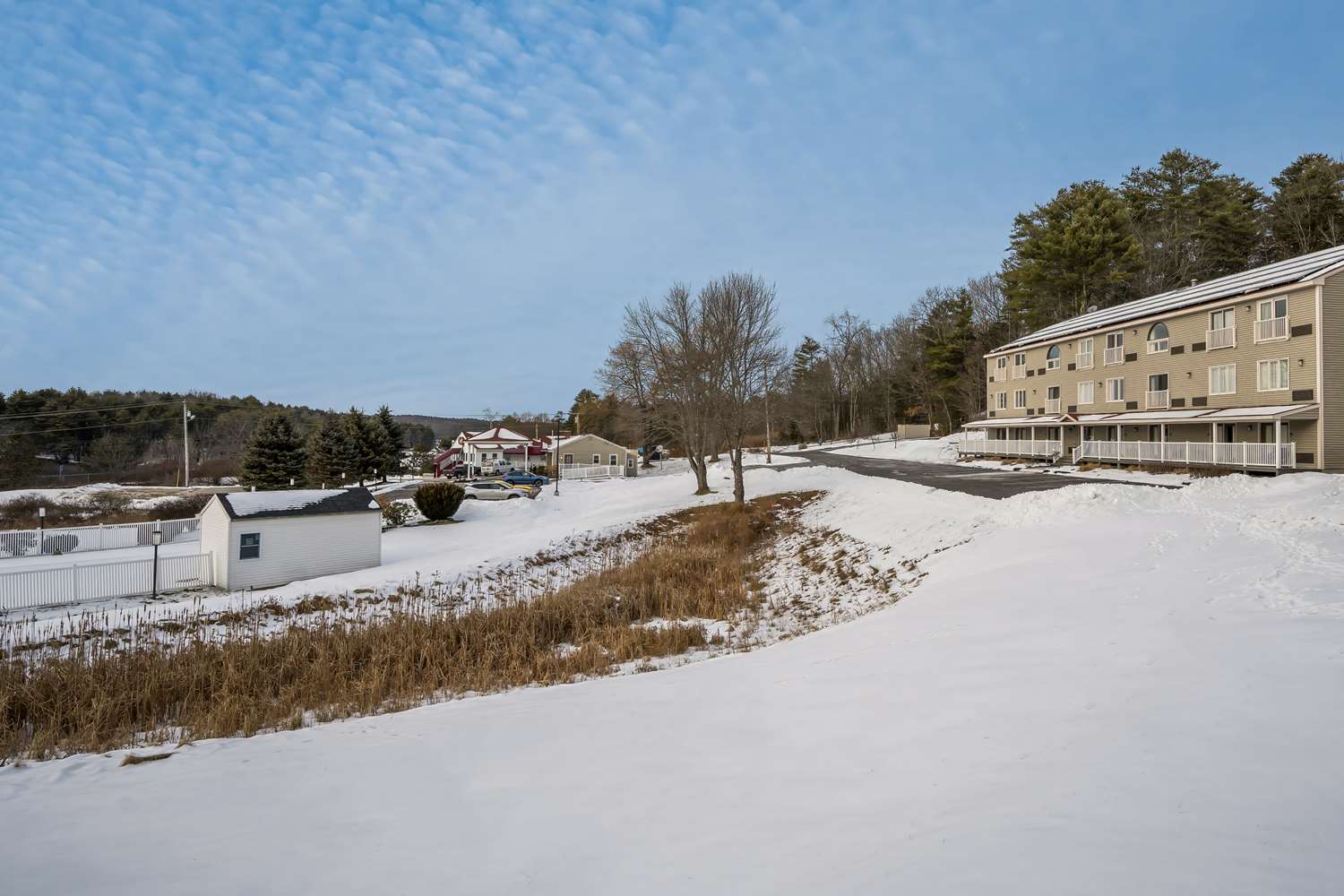The picture captures a serene wintertime scene dominated by a tan-colored, three-story building, potentially an apartment complex or hotel, situated in the back right corner. The building features multiple white-trimmed windows and railings, adding to its structured appearance. The foreground is a stark contrast of white, snowy land, interspersed with patches of brown winter grass. Towards the left side, a white shed with a single window and a white picket fence can be seen, adding quaint charm to the scene. The sky above is mostly clear with scattered clouds, allowing ample sunlight to brighten the landscape. Surrounding this central structure are leafless trees and a mix of other buildings, including homes, a barn, and a garage, with a few distant cars, some blue and gray or silver, visible near these structures. The middle of the image features a slightly elevated hill with rows of evergreen trees, providing a natural backdrop to the crisp, wintry tableau.